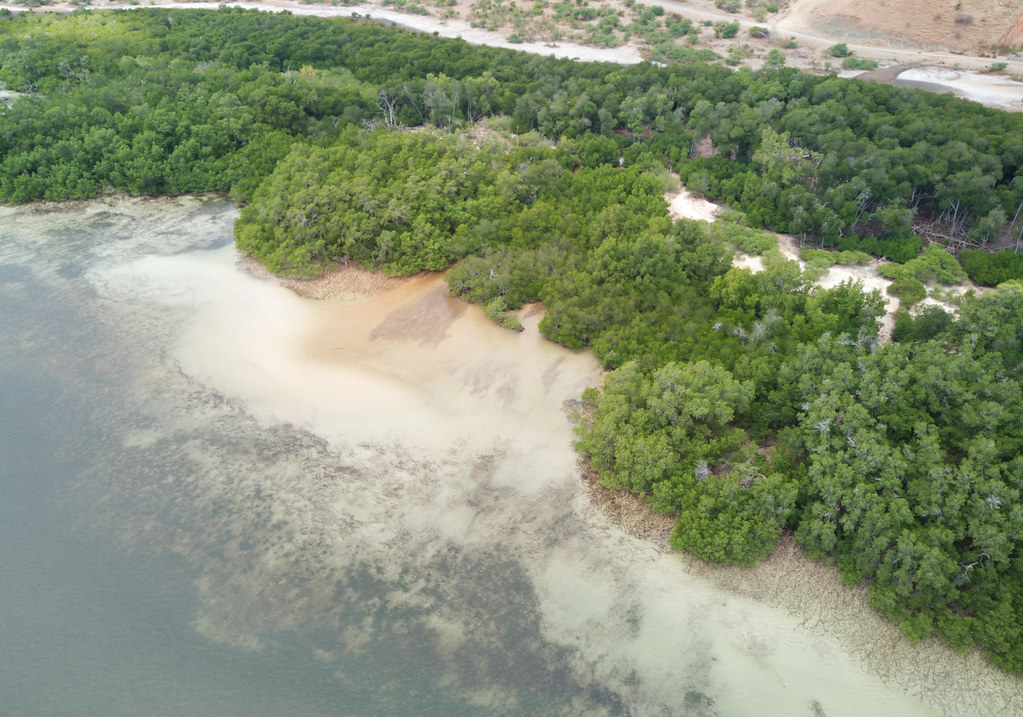This aerial view captures a diverse coastal landscape from approximately 200 feet in the air. The image prominently features a diagonal strip of sand running from the lower right to the upper left, flanked by foamy waves where the water meets the shore in the lower left corner. Over half of the scene is dominated by dense greenery, including full-grown trees, bushes, and patches of scrub brush interspersed with sandy dirt, indicative of an arid region. The treeline varies in density, with a particularly thick band of trees giving way to a second treeline farther inland. At the top right of the image, a faintly visible sandy area transitions into what appears to be a road, flanked by an arid, desert-like expanse. This detailed interplay of coastal elements and vegetation highlights the complexity and richness of the landscape in this almost-isometric perspective.